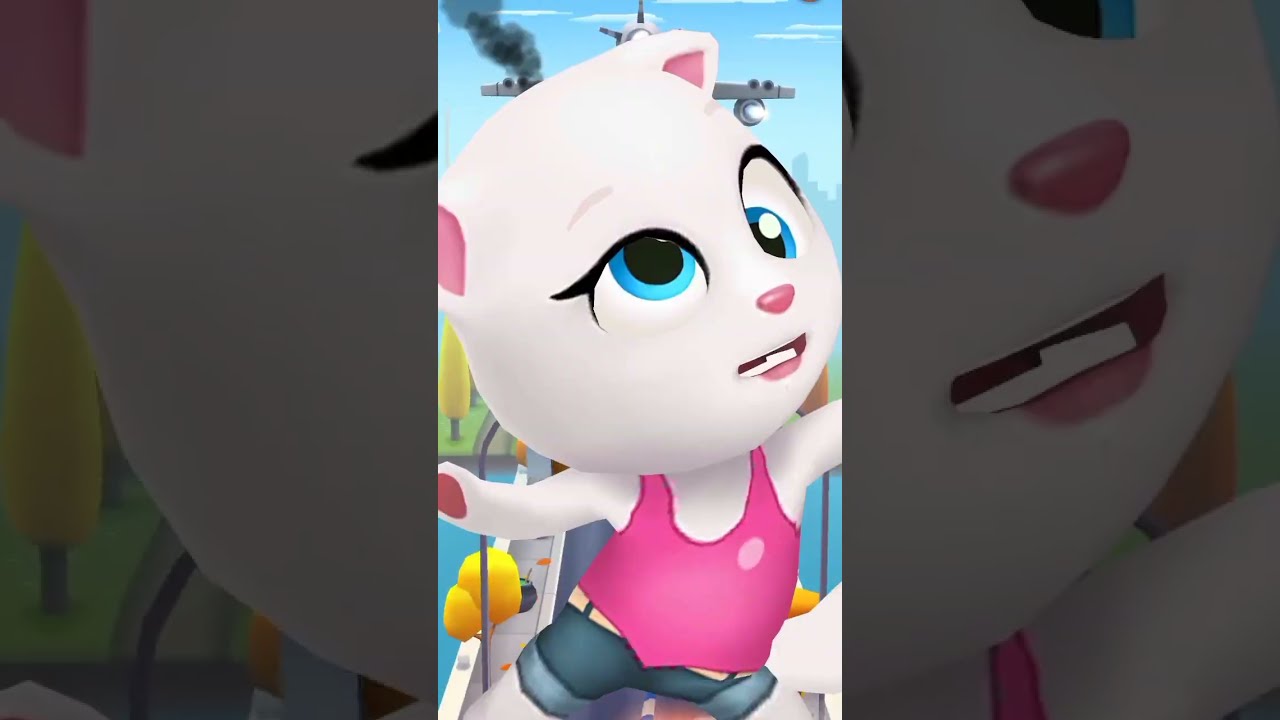The image appears to be a highly detailed scene from a cartoon or 3D animated movie, featuring an anthropomorphized white cat with distinctive blue, crossed eyes. The cat is dressed in a pink tank top adorned with a white logo, cuffed denim shorts with a white belt, and stands with its arms and legs splayed apart. It has pink palms, ears, and a cute pink nose, with a hint of teeth showing, which gives it a dazed or bemused expression. The background shows a white sky filled with feathery clouds, a distant large body of blue water, green and yellow trees, and a plane with gray smoke billowing from one of its engines. The overall setting is vibrant with colors of white, blue, pink, navy, yellow, gray, and green, suggesting an outdoor scene, possibly from a video game or animated show. The image is framed by grayed-out areas on both sides that emphasize the central vivid portion, drawing attention to the comedic and whimsical tone of the scene. The cat appears to be the central focus of the image, set against what seems to be a lively and potentially chaotic environment.